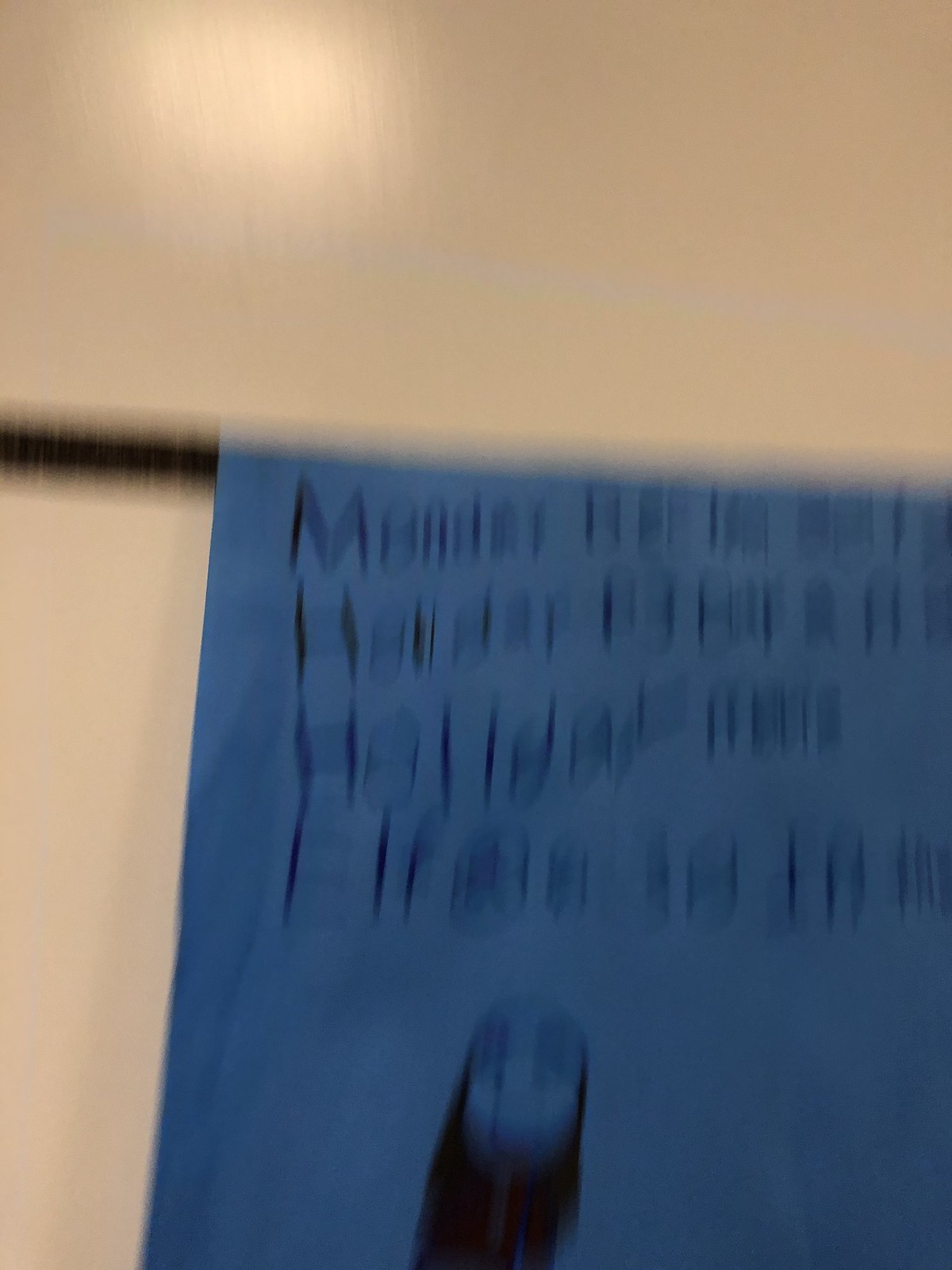This is a blurry photograph of a blue piece of construction paper set against a white wall. The image quality is poor, likely due to natural lighting creating an unfocused effect, akin to seeing without glasses. Despite the blurriness, one can discern four rows of uneven, childlike handwriting in capital letters. The first row seems to spell out "Monday," followed by other words that include "holiday," though the exact text is difficult to read. At the bottom of the paper, there is a drawing of a face with long black hair, along with some indications of eyes and a nose. This piece of art, seemingly created by a child, appears to be hanging on a wall. There's a noticeable bright light in the upper left corner of the image, contributing to the overall blur.